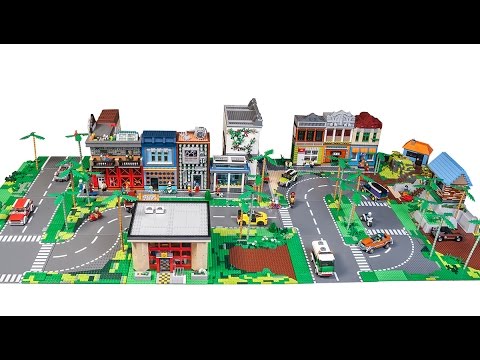The image depicts a vibrant and detailed LEGO toy city set on a white background, framed by black horizontal lines at the top and bottom. The miniature city includes an array of colorful buildings, roads, vehicles, and greenery, meticulously crafted to resemble a bustling town. 

The roads are gray with white dashed lines and marked crosswalks, weaving through the city and encircling a rotary filled with vehicles like cars, buses, and motorcycles in various colors, including red, green, yellow, blue, and orange. The ground areas representing grass are lush green, dotted with trees—some with yellow or white stems and green leaves—and patches of brown dirt.

In the upper right center of the image stands a cluster of three buildings, including a two-story hotel with a distinctive red roof. Nearby, palm trees and a tiki hut with a blue roof add a tropical touch, alongside a jeep. The upper left side features four buildings: one with white pillars and a blue roof, a two-story building with a red roof, and another with a dark blue roof. 

The bottom center showcases a prominent white building with a red entrance and a checkerboard walkway, bordered by green grass. Just behind it, a yellow car travels horizontally. Additional buildings, a mix of tan, red, blue, beige, and white structures, are spread throughout the background, characterized by varied architectural details like brown, gray, or blue roofs and white awnings.

This meticulously designed LEGO city portrays an intricate, colorful, and lively miniature urban landscape complete with various structures, vehicles, roadways, and greenery.